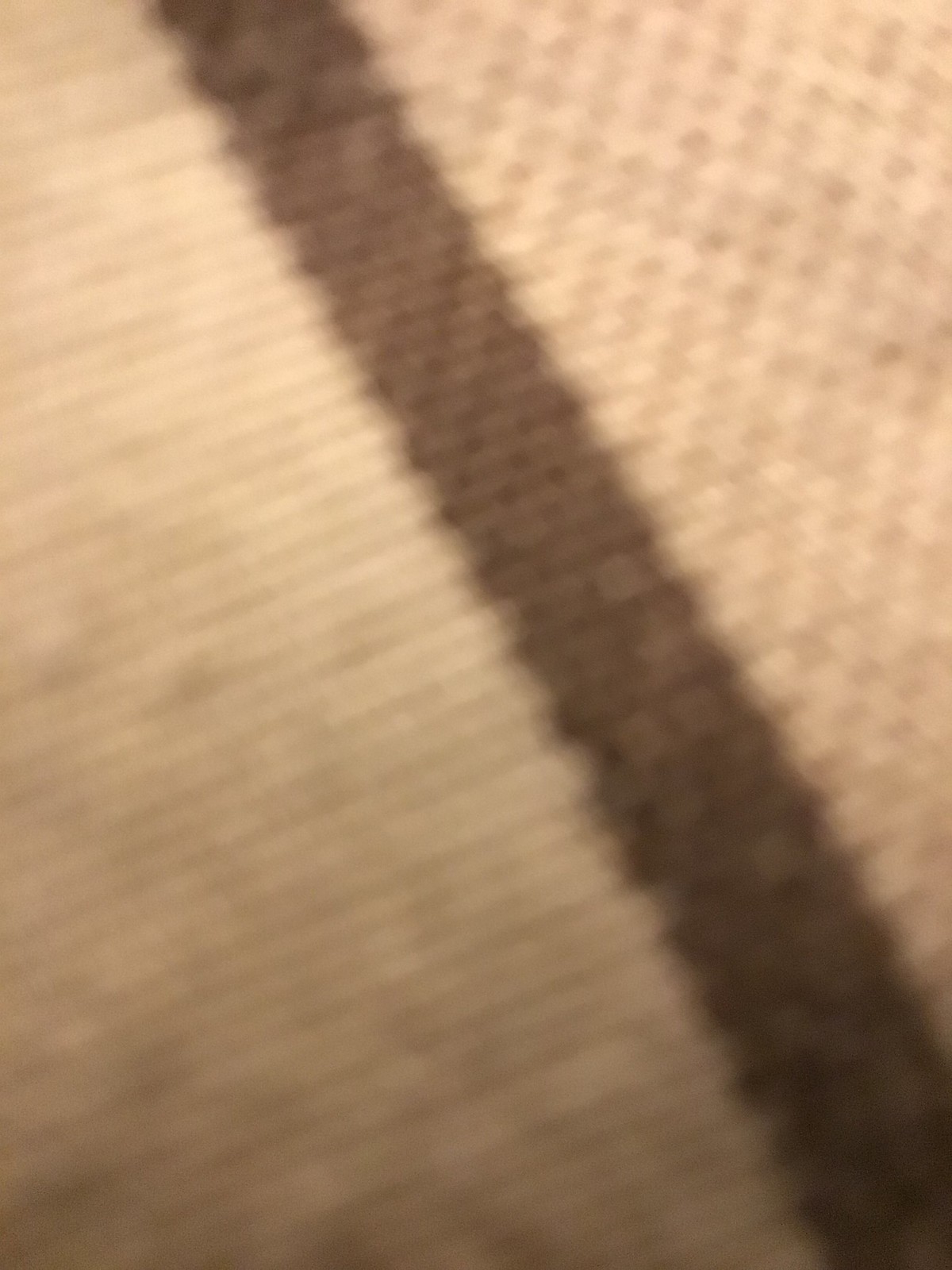The image showcases a brown, woven fabric mat featuring distinct color variations. On the left and right sides of the mat, there's a light brown hue, which converges into a thick, darker brown rectangle running down the center. Although the image is slightly out of focus, the texture and weave of the mat are still discernible. The mat might be part of a larger textile item, such as a blanket or a bag. Additional shading accents, including dark gray tones, are present at the bottom left and bottom right corners, enhancing the overall texture and visual interest of the piece.